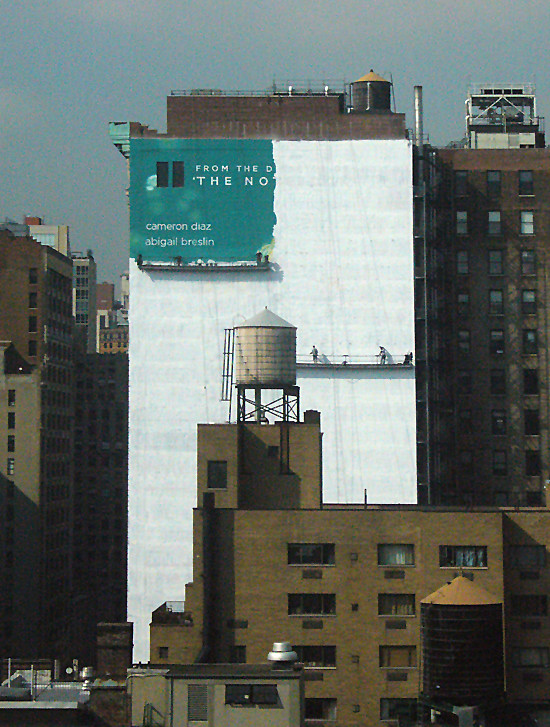In this urban landscape image, a blue-gray sky forms the backdrop for several buildings in the foreground. Central to the scene is a tall, white building extending nearly to the rooftop, where two workers are on brown scaffolds—one higher than the other—on either side. The men appear to be painting a billboard that partially reads "Cameron Diaz" in white letters, with other text like "from the" and incomplete words like "D" and "N O." The top portion of this sign has a greenish-blue hue. Below the white building, there is a shorter brown building with visible windows, and above it, a brownish tower capped with a lighter section and railings. Additional buildings of varying heights and colors flank the central structures, contributing to the city's varied architectural palette. To the forefront and left, a white water tower stands prominently above this eclectic assembly of urban structures.